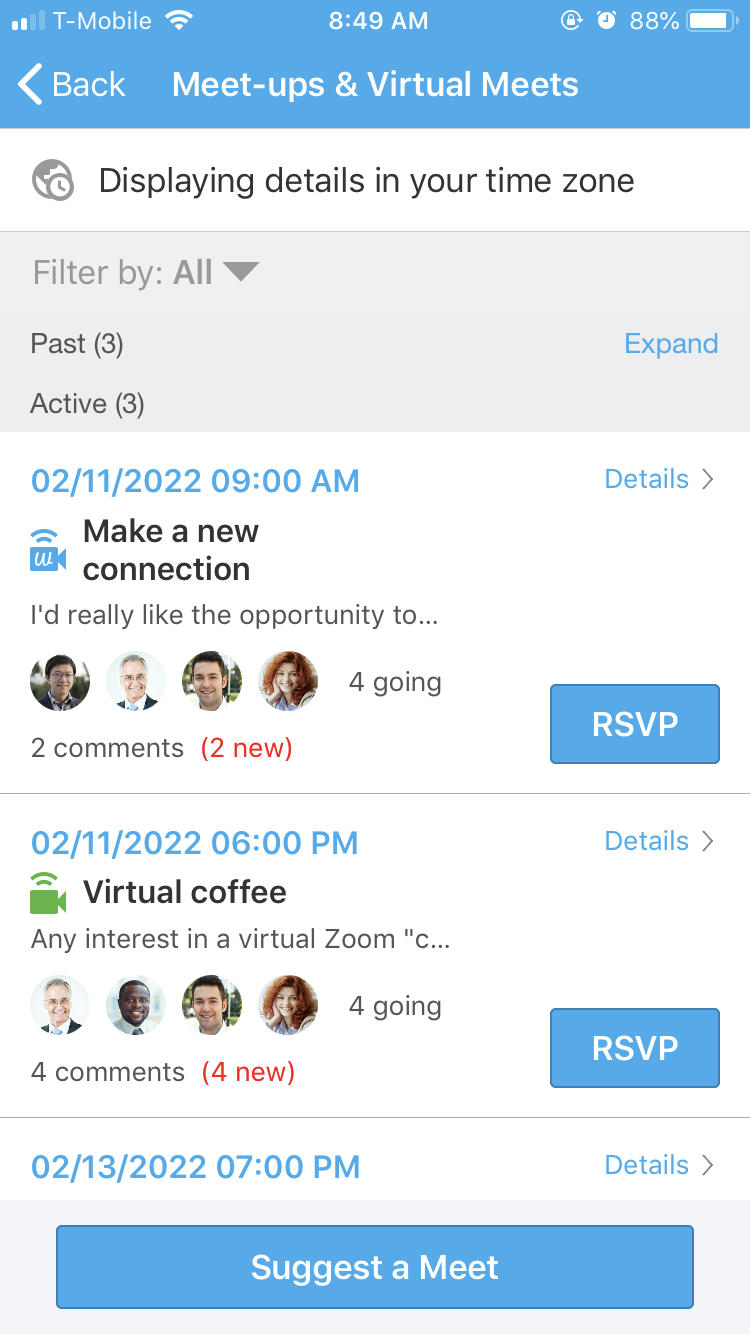The image depicts a mobile screenshot taken at 8:49 a.m., as indicated by the timestamp at the top. The device is on the T-Mobile network and shows a battery level of 88%. Below the status bar, a thin blue bar features white text that reads "Meetups and Virtual Meets," with a back option on the left side.

The background is predominantly white, displaying the message "Displaying details in your time zone" in black text. Directly beneath this message is a gray bar containing filter options: "Filter by: All," "Past (3)," "Active (3)," and an "Expand" option in blue text on the right.

Following the filter bar, two meetups are listed. The first meetup is scheduled for February 11, 2022, at 9:00 a.m., titled "Make a New Connection." A brief description follows, ending with an ellipsis. Four attendees are shown via headshots, with two comments underneath, denoted by "(2 new)." A blue "RSVP" button is situated to the right.

The second meetup is also on February 11, 2022, but at 6:00 p.m. It is advertised as a "Virtual Coffee" event, with the text "Annie interested in virtual Zoom." The same four attendees are shown, suggesting duplicated headshots. This meetup has four comments, noted by "(4 new)," and another blue "RSVP" button on the right.

At the bottom of the screen is a prominent blue button labeled "Suggest a Meet" in white text.